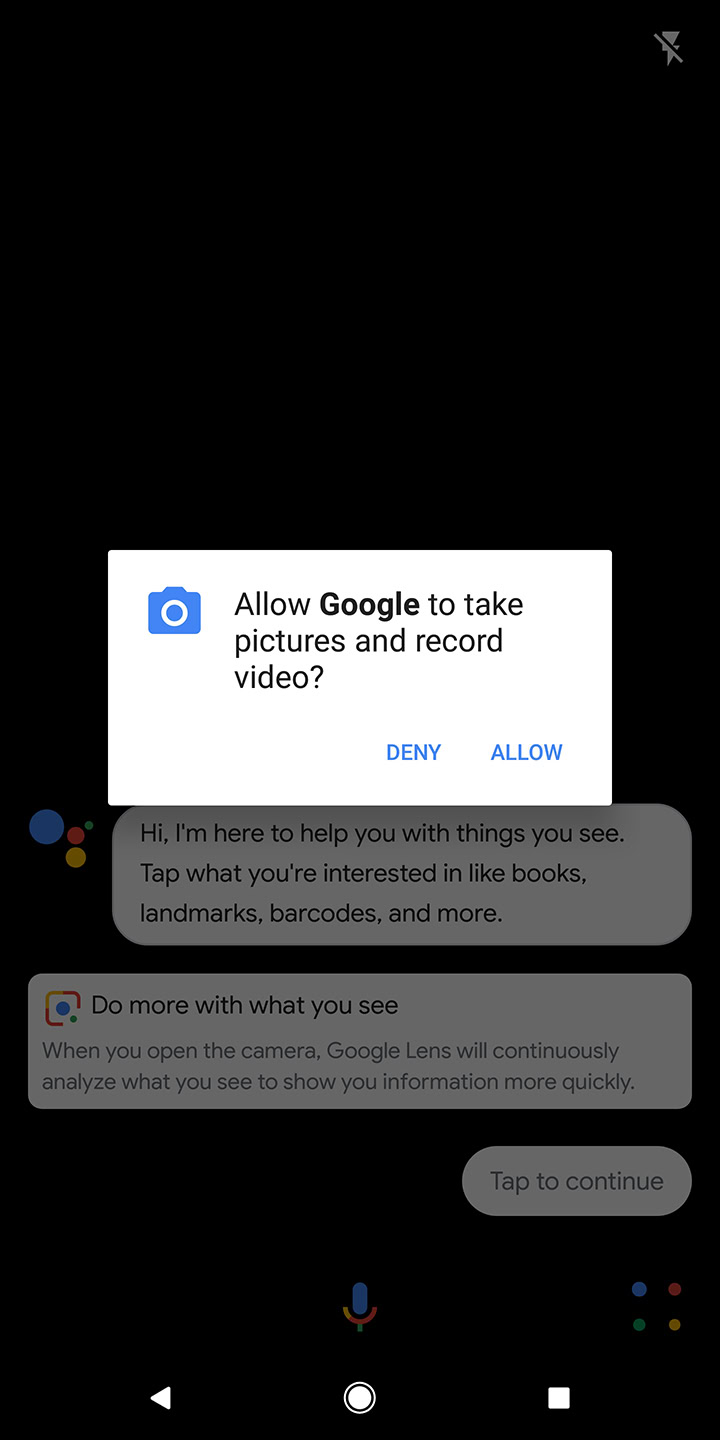The image is a screenshot of a smartphone displaying a pop-up notification asking for permission to allow Google to take pictures and record videos. The notification is accompanied by a camera icon and offers two options: "Deny" or "Allow." The background screen, which is dimmed behind the pop-up, presents a message from Google Lens: "Hi, I'm here to help you with things you see. Tap what you're interested in, like books, landmarks, barcodes, and more." Below this message, there's a button labeled "Do more with what you see."

Further instructions indicate that when you open the camera, Google Lens will continuously analyze your surroundings to provide you with relevant information quickly. There is a prompt encouraging the user to tap to continue. Essentially, to utilize Google Lens's feature of identifying objects, giving information, or assisting with various tasks, the user must grant Google permission to access the camera by selecting the "Allow" option.